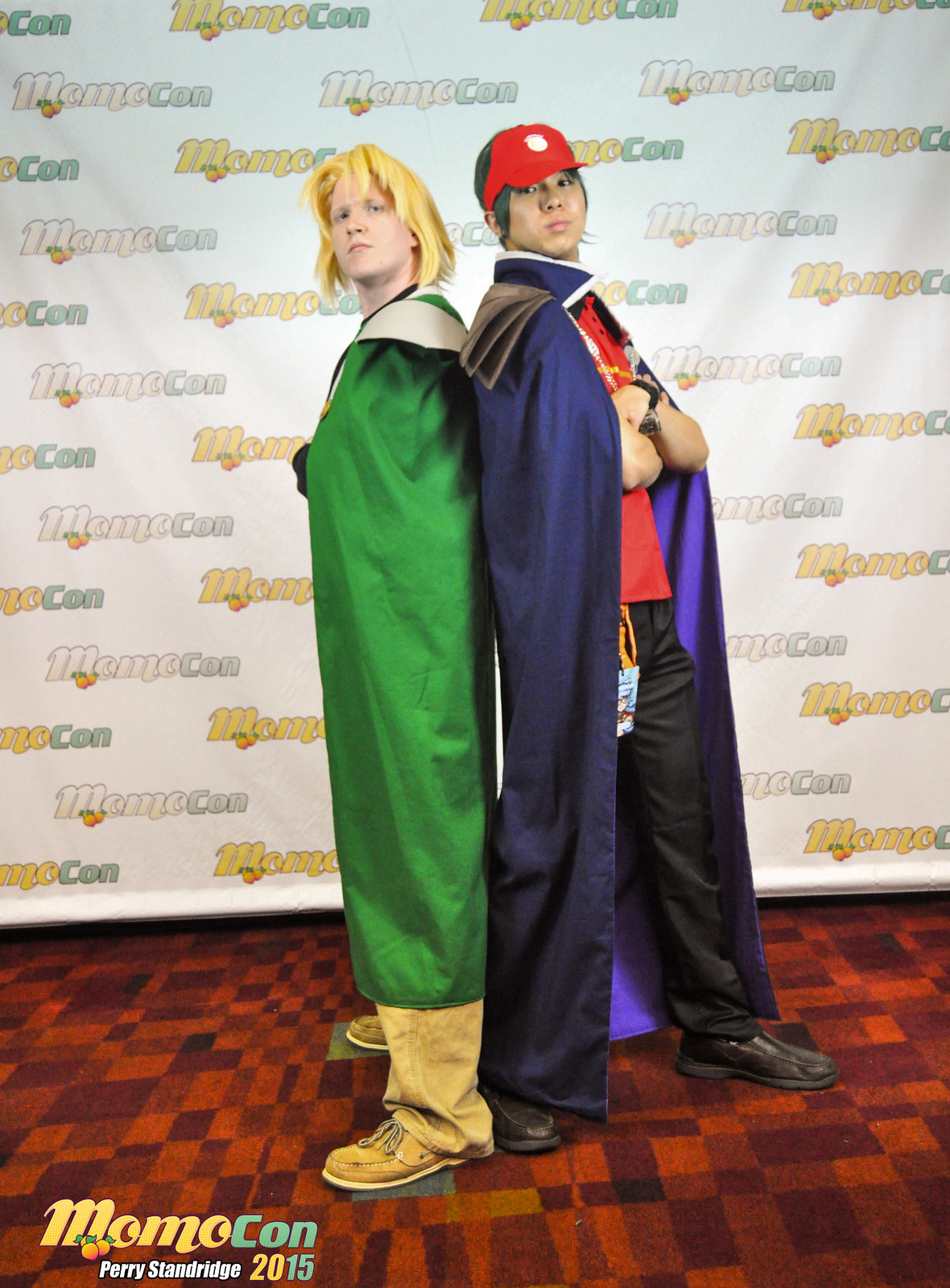This image, taken by Harry Stan Ridge in 2015 at MomoCon, features two individuals posing in a back-to-back stance, attempting to look tough. They are cosplayers dressed as characters from popular media. The individual on the left, a white person, is dressed as Link from The Legend of Zelda, complete with a blonde wig, green robe, green cape, and boots. The person on the right, potentially Asian, is wearing a red hat, a dark blue (or perhaps purple) cape, black pants, and a red shirt with a cross on it, reminiscent of a character from an anime. The background features a MomoCon banner with a faded orange-green gradient and peach icons, alongside the text "Perry Standridge 2015" in the bottom left corner.